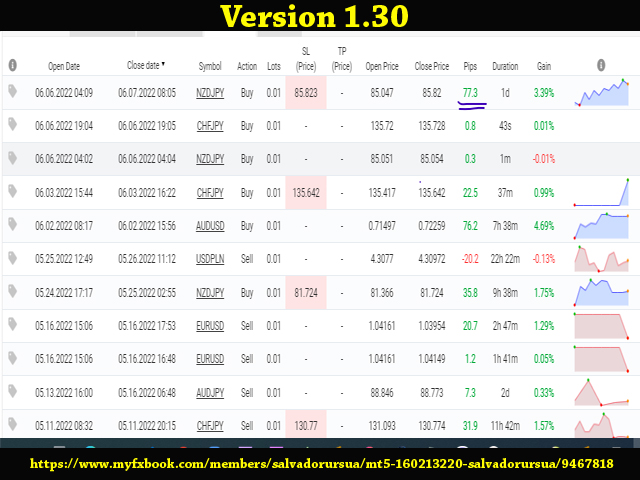This portrait-oriented screenshot features a comprehensive trading log from the website www.myfxbook.com/members/salvadorursua/mt5 (with additional identifying numbers). It is prominently labeled "Version 1.30" in bold yellow text across a black stripe at the top.

The chart is meticulously detailed, containing 14 columns under a well-defined header, which includes (from left to right): an information icon (I in a circle), Open Date, Close Date (with a drop-down menu), Symbol, Action, Lots, SL (price), TP (price), Open Price, Close Price, PIPS, Duration, Gain, and another information icon (I in a circle).

Highlighted in the first row of the chart, the recorded trade details are particularly emphasized. Key information includes: 

- **Open Date**: June 6, 2022, at 4:09
- **Close Date**: June 7, 2022, at 8:05
- **Symbol**: NZDJPY
- **Action**: Buy
- **Lots**: 0.01
- **SL Price**: $85.823 (highlighted within a pink box)
- **Open Price**: $85.047
- **Close Price**: $85.82
- **PIPS**: 77.3, underlined twice in blue ink
- **Duration**: 1 day
- **Gain**: $3.39

To the far right, a small visual chart depicts the trade's progression, illustrating a rise from the bottom to the top in red. Handwriting annotations appear on the image, indicating a personal touch from the creator, who appears keen to highlight the trade's successful PIPS gain.